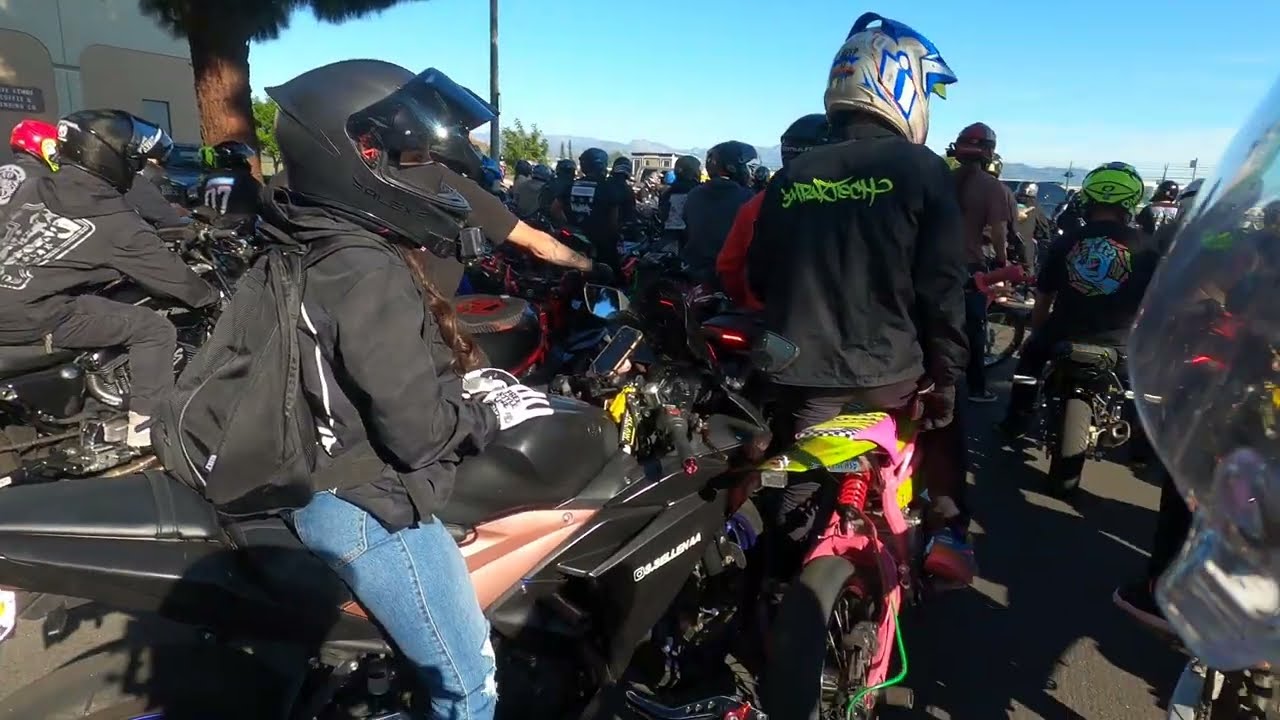The photograph captures an outdoor scene at what appears to be a biker rally or meeting. The perspective is from behind a large group, primarily showing the backs of around 50 bikers. These riders, dressed predominantly in black or dark sweatshirts and jackets, are wearing helmets of various colors, including green, blue, and white. The bikers are either sitting on their motorcycles or standing beside them, all facing towards something indistinct in the upper right corner of the image.

The scene takes place on some sort of pavement, partially visible in the bottom left corner. The nearest individual to the camera sports a black helmet, a dark jacket, blue jeans, and a backpack, with white gloves on their hands. Nearby, another person is seen with a black jacket adorned with green writing, and there's mention of someone wearing a black hoodie with white accents.

In the background, the setting includes mountains or hills and a tree close to a building, providing depth to the photograph. The sky above is a vivid blue with a few clouds scattered across the horizon, which appears almost white. There's a large tree on the upper left side of the image, basking in sunlight.

A glass object on the right side of the image is somewhat mysterious, but it could potentially be a motorcycle windshield. The overall impression is one of anticipation, with the bikers seemingly poised to set off, unified in their forward gaze.